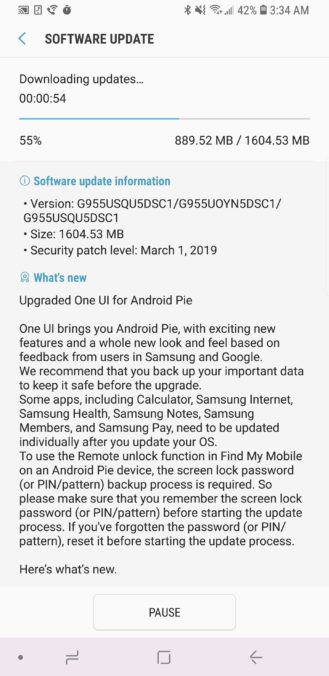The image captures a smartphone screen displaying a software update in progress. At the top of the screen, the user interface showcases various status icons indicating Wi-Fi connectivity, signal strength, a battery level at 42%, and the current time as 3:34 AM.

Just beneath these icons, a header reads "Software Update." Below this header, there is a progress section that features a timer showing "00:00:54" and a blue progress bar indicating 55% completion, as noted at the bottom left. To the right of the progress bar, it shows the data transferred: "889.52 MB / 1604.53 MB."

Further down, a gray information box provides detailed software update information:
- Version: G955USQUIDSC1 / G955UOY95DSC1 / G955USQU5DSC1
- Size: 1604.53 MB
- Security Patch Level: March 1st, 2019

The "What's New" section lists "Upgraded One UI for Android Pie," and includes a burst graphic to highlight this update. The accompanying text elaborates that "One UI brings you Android Pie with exciting new features and a whole new look and feel based on feedback from users in Samsung and Google." Users are strongly encouraged to back up their important data before proceeding with the upgrade. Specific instructions are provided for app updates post-upgrade, including for Calculator, Samsung Internet, Samsung Health, Samsung Notes, Samsung Members, and Samsung Pay. Additionally, for functionalities like "remote unlock" and "Find My Mobile" on an Android Pie device, the screen lock password (PIN/pattern) backup process is mandatory.

A small white pause button rests beneath this detailed explanation. At the bottom of the screen, the phone's navigation bar is visible, featuring symbols for a dot, two lines indicating opposite directions, a square, and a left-pointing arrow.